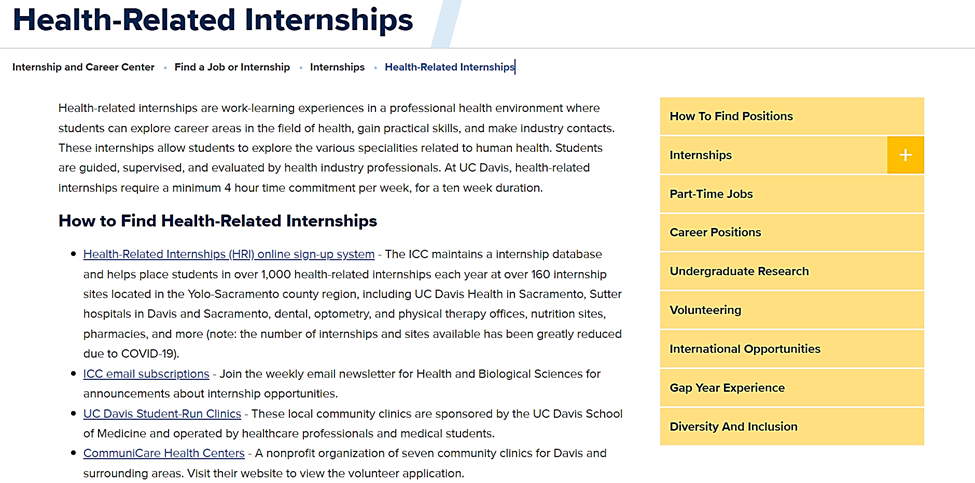In this image, a webpage is displayed prominently featuring information about health-related internships. At the top of the page, the title "Health Related Internships" appears in bold black text. Below the title, a navigation path is outlined showing: Internship and Career Center > Find a Job or Internship > Internships > Health Related Internships, with the final link highlighted in blue.

Beneath the navigation path, a paragraph in black text describes health-related internships as work-learning experiences in professional health environments. It elaborates that these experiences allow students to explore various career areas within the field of health, gain practical skills, and establish industry contacts. The internships provide students with opportunities to delve into multiple specialties related to human health. They ensure students are guided, supervised, and evaluated by professionals in the health industry. Specifically, at UC Davis, health-related internships require a commitment of at least four hours per week over a 10-week period.

Further down, a section titled "How to Find Health Related Internships" appears in black text. Below this heading, four links are highlighted in blue: "Health Related Internships, HR Online Sign-Up System," "ICC Email Subscriptions," "UC Davis Student-Run Clinics," and "CommuniCare Health Centers."

On the right-hand side of the image, against a very light orange background, nine horizontal rows categorize additional resources. These categories include: "How to Find Positions," "Internships," "Part-Time Jobs," "Career Positions," "Undergraduate Research," "Volunteering," "International Opportunities," "Gap Year Experience," and "Diversity and Inclusion."